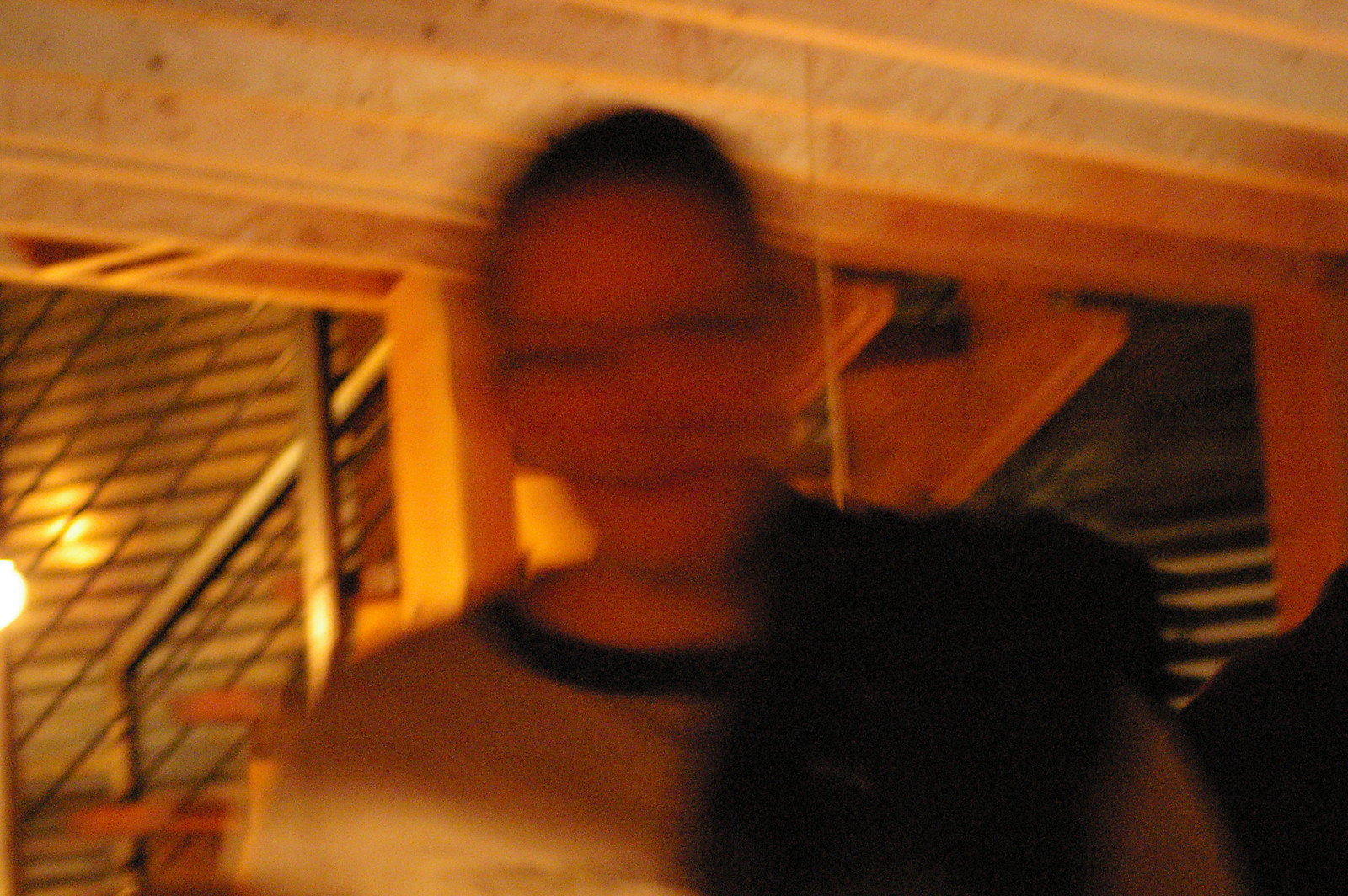In this blurry photograph, the subject appears to be a man situated indoors. He sports a shirt with a rounded neckline and a distinct black collar, the shirt itself being a blend of white and gray tones. Draped over his left shoulder, there is a dark-colored item, likely a jacket. His hair is cut short, and he has fair skin. The background seems to depict a warehouse-style loft, featuring wooden stairs with a metal handrail, a metal door, and a hanging bulb light emitting a warm yellow glow.